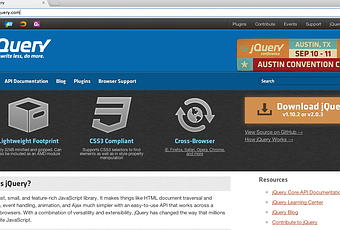The image is a cropped screenshot of a mobile browser displaying the jQuery website. The cropping excludes the extreme left and right sides of the webpage, revealing only a portion slightly left and right of center. The header of the webpage is in blue, featuring the white jQuery logo at the top left. To the right of the logo, a banner is present, consisting of an orange box with "jQuery" written inside, and adjacent to it, a blue and white box. The blue section of the box indicates "Austin, Texas," and the white section beneath it states "September 10th-11th." Below, partially cropped, are the words "Austin Convention," indicating the Austin Convention Center.

Directly underneath the header is a darker blue navigation bar displaying four categories: API documentation, blog, plugins, and browser support. Some additional categories are likely cut off. Further right, part of a search bar is visible. Below this navigation bar, three large gray icons are visible, each accompanied by a brief description. The first icon on the left is a box with the text "Lightweight Footprint" beneath it. On the far right, a prominent orange bar displays the text "Download jQuery."